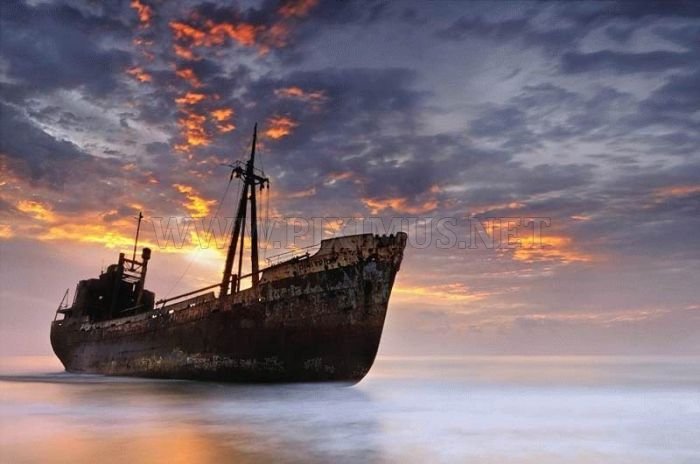The image depicts a large, rusted, and dilapidated old ship, reminiscent of an ancient pirate vessel, stranded in what appears to be shallow water, likely on a sandbar, in the middle of the ocean. The ship is positioned slightly off-center to the left, facing towards the right corner of the photograph. The colors of the ship and surrounding scenery include varied shades of brown, rust, gray, and orange. A thick mist hovers above the water, adding an air of mystery to the scene. Above, a stunning sky painted in hues of orange and blue, with gray and purplish clouds, suggests an impending sunset, casting limited yet vibrant light across the image. The only text visible is a watermark reading "www.pyximus.net."